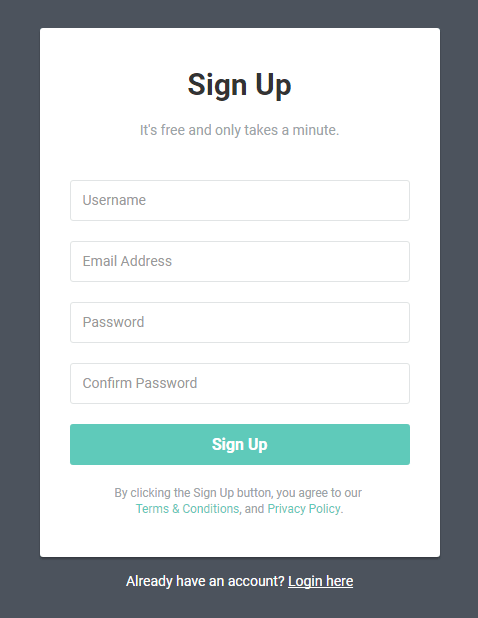The image depicts a vertically elongated black rectangle, on top of which sits a similarly elongated white rectangle, allowing a visible border of the black background. The bottom border of the black rectangle is slightly thicker than the top.

At the top center of the white rectangle, the text "Sign up" is prominently displayed. Directly above this, in smaller gray text, it says "It's free and only takes a minute." Below the "Sign up" text, there are four data fields arranged vertically:

1. The first field is labeled "Username" in gray text.
2. The second field, directly below the first, is labeled "Email Address" in gray text.
3. The third field beneath the second is labeled "Password" in gray text.
4. The fourth field, positioned below the third, is labeled "Confirm Password" in gray text.

Under these fields is a green "Sign Up" button that spans the same width as the data fields, with "Sign Up" written in white text on it. 

Beneath the button, a gray-colored text states, "By clicking the Sign Up button, you agree to our terms and conditions and privacy policy," where "terms and conditions" and "privacy policy" are clickable links highlighted in green.

At the very bottom, against the black background, there is white text reading, "Already have an account? Log in here," with "Log in here" underlined in white, indicating it as a clickable link.

The color palette includes black, white, gray, and green, suggesting that this is a segment of a website's sign-up form rather than the entire webpage.